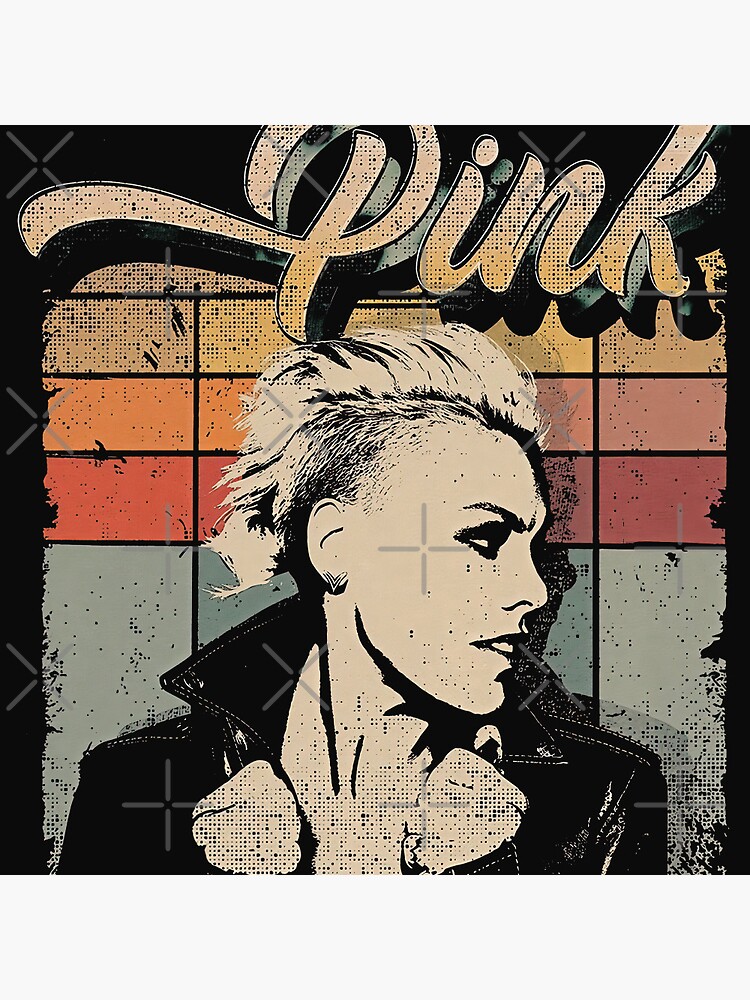The image features the iconic musical artist Pink, prominently labeled with her name in large, curly letters that transition from pink to orange hues. This vibrant text sits against a black backdrop dotted with a myriad of small points, giving it a gritty texture. Pink's portrayal is in dramatic black and white, evoking a striking cartoon-esque aesthetic. She stands in a side pose, turning her head to the right, showcasing her thick eye makeup and bold lipstick. Her hair is short, spiked back, likely blonde, and she sports a V-shaped earring. Pink is clad in a black leather jacket with the collar turned up, her hands possibly clenched into fists or adjusting the collar. The background is adorned with rectangular and square color blocks in shades of light blue, pink, yellow, orange, and red, interspersed with gray X's and crosses that give the image a layered, dynamic feel, reminiscent of fan art or merchandise from her concerts.